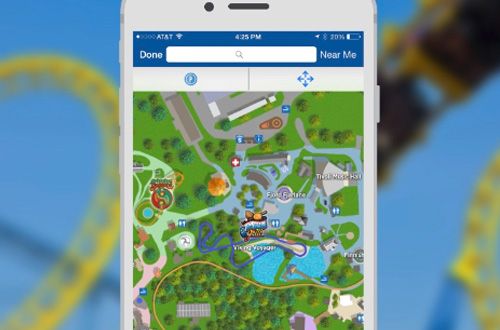A smartphone displays a video game map, indicating the game status as "Done" and "Near Me" at the top. The screen shows a vibrant gaming landscape featuring trees, rivers, and various buildings. The phone, connected to the AT&T network, shows the time as 4:25 p.m. and the battery level at 29%. In the background, a blurred blue sky and what appear to be roller coasters are visible, adding a sense of outdoor excitement. The front-facing camera and speaker are located at the top of the phone, while the power button is positioned on the right side, and the volume keys are on the left.